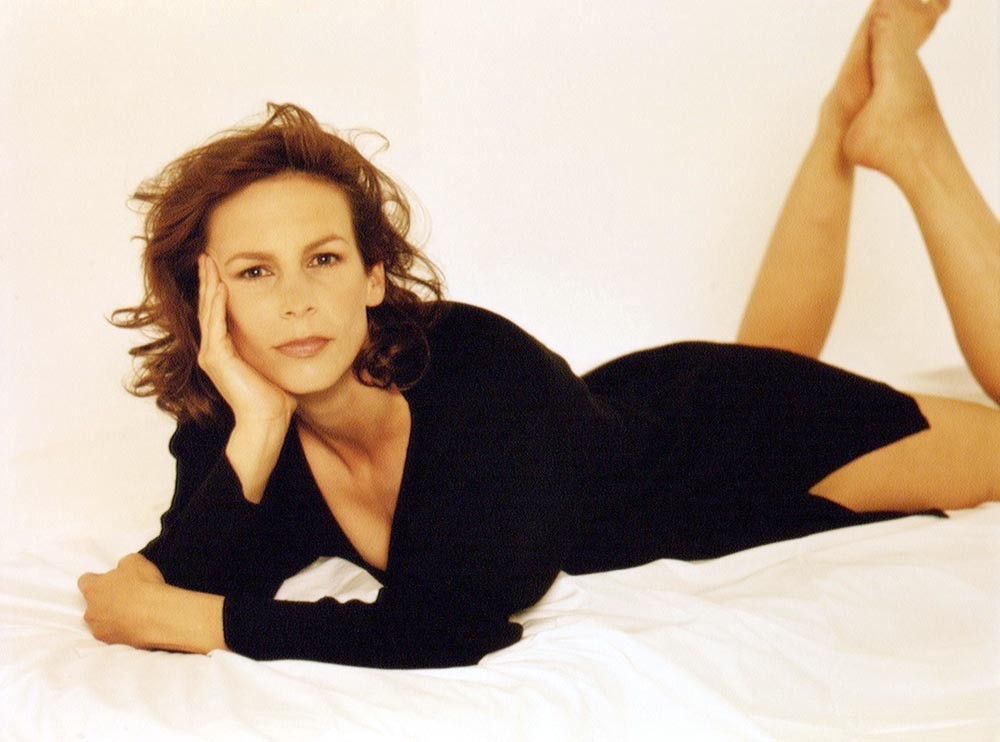In this professional photograph, a young Jamie Lee Curtis is captured laying stomach-down on a bed with her legs playfully raised behind her. She is dressed in a fitted black dress with long sleeves. Her posture suggests a relaxed yet poised demeanor, with her right hand resting under her chin and her left hand supporting her on the bed. Her wavy hair, a dark red to light brunette shade, cascades down to her shoulders, framing her face. Jamie Lee Curtis's expressive brown eyes are fixed directly at the camera, creating a captivating and intimate gaze. The background features an off-white, cream-colored wall with no adornments, emphasizing the simplicity and elegance of the setting. The bed’s sheets are wrinkled and of a similar white or cream hue, complementing the overall minimalistic aesthetic of the image.